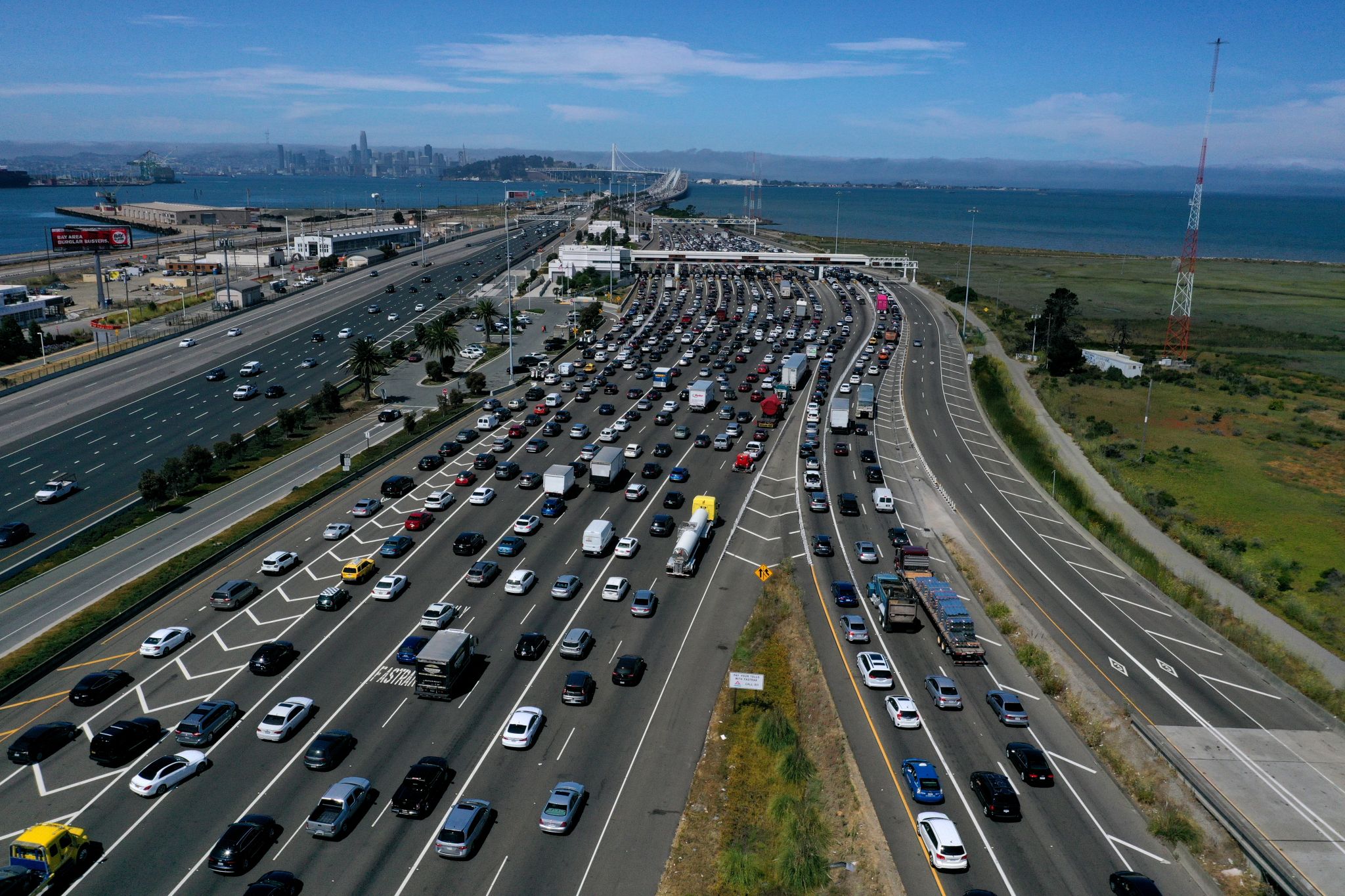Aerial view of a bustling multi-lane freeway system, featuring at least a dozen lanes teeming with vehicles. The traffic flows towards a distant toll booth. The horizon showcases a body of water with another city dotted with tall buildings. The skyline is a serene light blue, accentuated by puffy white clouds. To the right of the freeway, lush trees and grass border the road, alongside a prominent red and white steel tower. On the left, an industrial area with gated sections and a port is visible. Beyond a barrier, another section of the freeway with sparse traffic heads towards the camera. The intricate network of roads and varied landscapes create a dynamic and detailed urban panorama.